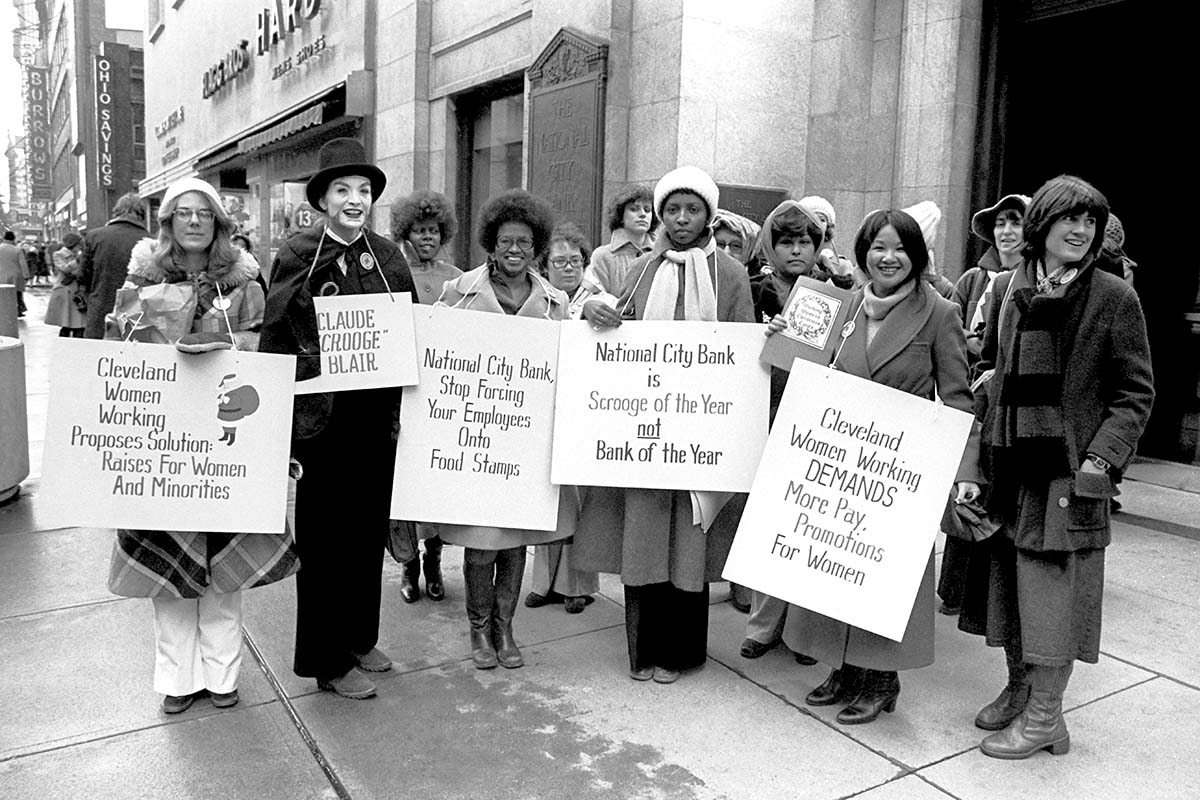This black-and-white photograph, likely from the 1960s or 70s, depicts a diverse group of predominantly feminine-presenting individuals at a protest on a cold day, as evidenced by their heavy coats and scarves. In the foreground, seven people hold various protest signs, while a crowd gathers in the background. Starting from the left, the first sign carried by a Caucasian woman with glasses and a white beanie reads, "Cleveland Women Working Proposes Solution: Raises for Women and Minorities." Next to her, a man dressed as a circus mime in a black coat and stovepipe hat holds a sign saying, "Claude Scrooge Blair." Continuing, an African-American woman with glasses and an afro displays a sign that states, "National City Bank - Stop Forcing Your Employees Onto Food Stamps." Another African-American woman in a white beanie and large scarf stands next, her sign declaring, "National City Bank is Scrooge of the Year, Not Bank of the Year." To her right, an Asian woman smiling broadly holds a smaller, illegible plaque in her hand and wears a sign around her neck that reads, "Cleveland Women Working Demands More Pay, Promotions for Women." The group appears unified in their message against National City Bank, advocating for better working conditions and fair pay for women and minorities.